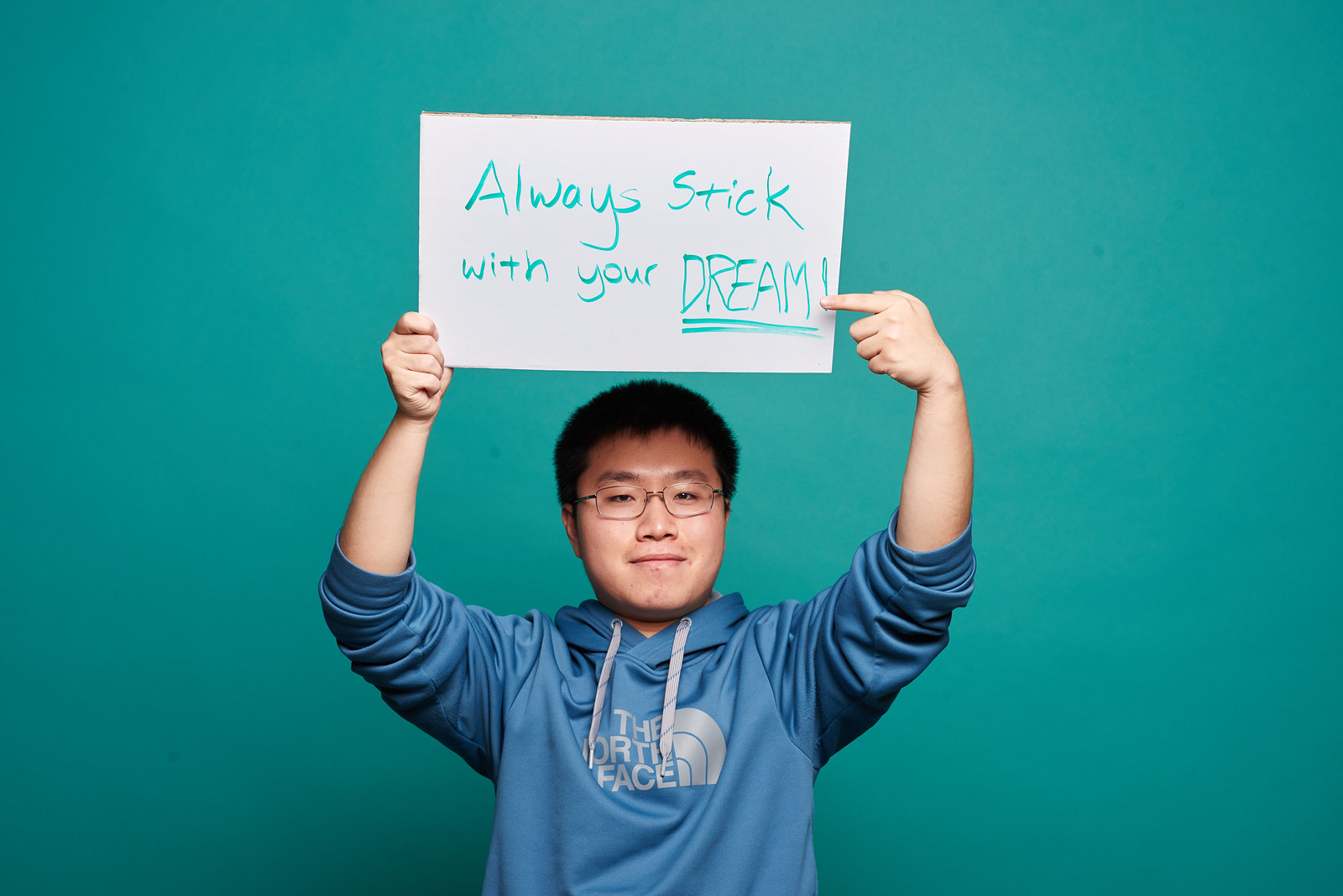The photograph captures a young Asian man, around 22 years old, holding a white cardboard sign above his head. The sign, approximately 12 by 7 inches, is handwritten in green or teal ink and reads "always stick with your DREAM!" The word "DREAM" is emphasized in capital letters, underlined twice, and followed by an exclamation point. He points to the word "DREAM" with his left hand. The man is wearing a long-sleeved, powder blue North Face hoodie with gray ties, distinct for its brand logo on the chest. His sleeves are rolled up to his elbows, and he sports short black hair and thin, rectangular, brown-rimmed glasses. He has a slightly rectangular face with a subtle, closed-mouth smile. The background wall matches the teal color of the text on the sign, creating a harmonious color coordination in the photo.